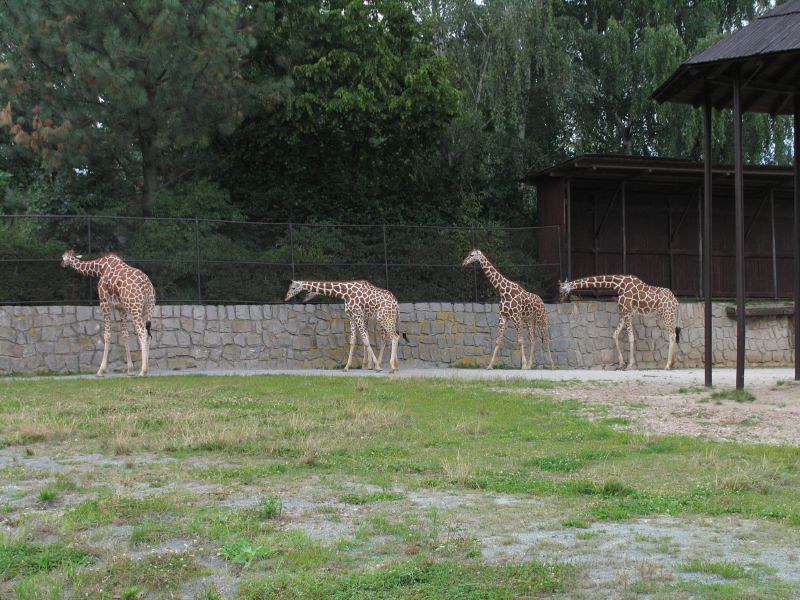This outdoor zoo photograph captures a scene of five giraffes inside an enclosure, with four giraffes clearly visible and a fifth partially hidden behind the second giraffe. The giraffes, wearing their distinctive tan skin adorned with chocolate brown spots, stand separately with their heads angled variably, all looking towards the left. The enclosure is framed by a stone wall, mottled gray with patches of moss adding touches of brown and green. Behind the wall, tall dark green trees and a lush background of foliage enhance the natural setting. 

In the right portion of the image, there is a shaded area supported by long cylindrical black pipes and topped with a black roof, likely providing shelter for the giraffes. Additionally, there is a small dark brown wooden shack without doors visible. The ground within the enclosure is a mix of light green grass with some trampled tan and gray patches. The sky above is cloudy, casting a diffuse light over the scene, with colors in the photograph including hints of cyan, green, brown, white, gold, and yellow.